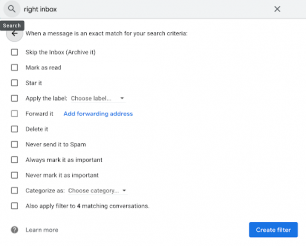This image displays an interface featuring a search bar at the top, containing the typed text "inbox." Below the search bar, several text options and commands are visible. These include a "Back" button and instructions for handling emails that exactly match the search criteria. The options listed are: skip the inbox, archive it, mark as read, star it, apply a label (with a prompt to choose a label), forward it, delete it, never send it to spam, always mark it as important, never mark it as important, categorize it (with a prompt to choose a category), and also apply the filter to matching conversations. At the bottom right corner, there is a "Create filter" button. None of the options have been selected yet.